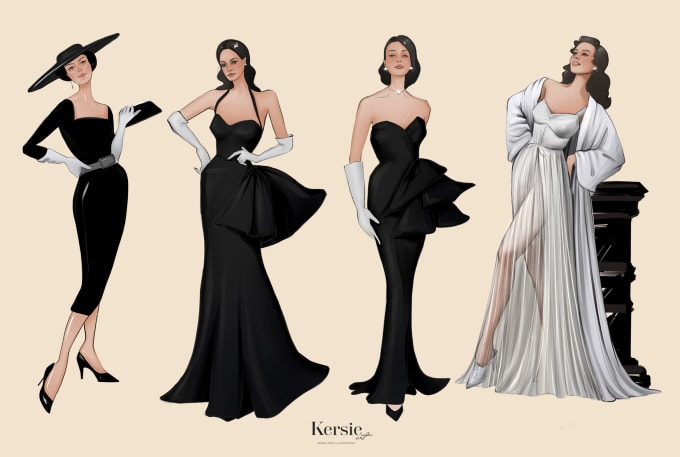This rectangular art piece, measuring approximately 5 inches wide and 3 inches high, features a detailed and elegant illustration of a tall, thin woman of Caucasian descent with dark black hair drawn four times, each in a different exquisite outfit and pose. Set against a light peach background, the artwork showcases the woman's versatility and the beauty of the dresses she's modeling, likely designed by "Kersie," as indicated by the text at the bottom of the image.

On the far left, the woman is adorned in a sophisticated ensemble with a wide-brimmed hat, her hair styled into twin buns. She wears a black, long-sleeved dress that falls just below her knees, paired with white gloves, black high heels, and a small black handbag. The dress features a square neckline, adding a touch of classic elegance.

The second depiction presents her with her hair down, donning a black halter-top dress that extends to the floor, concealing her feet. She again sports white elbow-length gloves, emphasizing a timeless grace.

In the third section, her hair is side-parted, complemented by pearl earrings. She wears a strapless, mermaid-fit black dress that hugs her form and flows to the ground. The familiar white gloves enhance her poised look.

On the far right, the woman is illustrated in a more relaxed, yet equally stylish, posture. She leans back against a podium, head tilted upwards, in an all-white ensemble that resembles a nightdress with a matching bathrobe. The bottom of her dress is semi-transparent, revealing her legs and white shoes, adding a modern, airy feel to the composition.

Overall, this image captures the elegance and variety of the dresses, as well as the sophistication of the model, presenting "Kersie" as a distinguished designer.